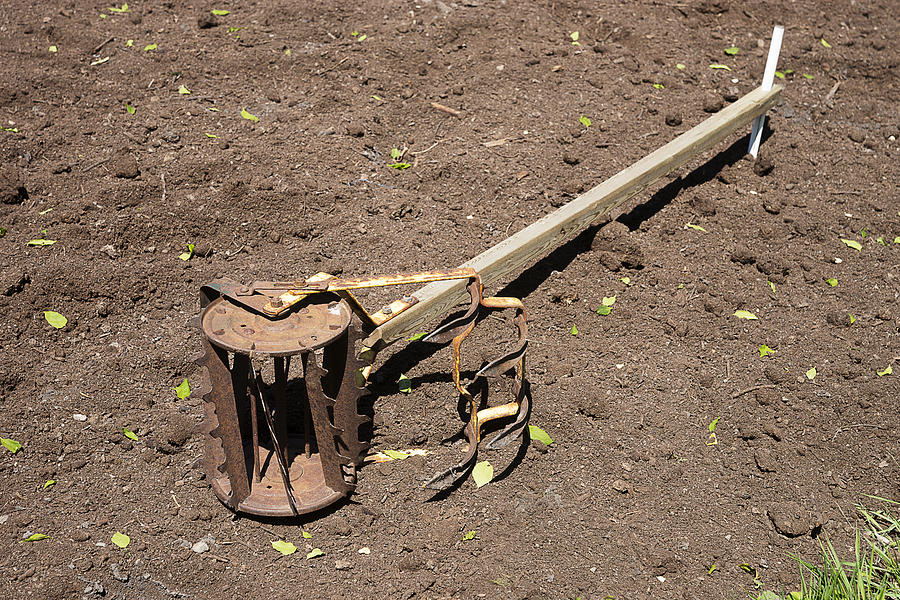The vibrant outdoor photograph vividly captures a vintage gardening tool, most likely a cultivator, lying diagonally in the middle of a dirt field. The tool features a long, aged wooden handle with a smaller white piece of wood driven through it to form a handle. The metal components at the bottom are heavily rusted, indicating significant use and age. The cultivator showcases a round, toothed design for tilling soil and a clawed section that can be adjusted for different positions. Scattered green leaves are strewn around the soil, providing a contrast to the primarily brown dirt. In the bottom right corner, a small patch of green grass subtly indicates the edge of the field. The image is well-lit, presenting a clear and detailed view of the tool against the soil, emphasizing its rustic character in the bright outdoor setting.